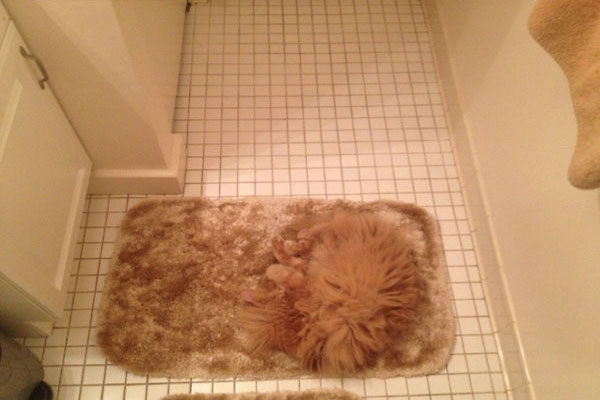The image depicts a bathroom floor with small, white tiles that have unbuffed, dirty brown grout between them. To the left of the frame, there is a white cabinet. The focal point is a shaggy bathmat, yellowish tan in color, positioned centrally. The bathmat appears untidy, as if it has seen better days, with a fluffy cat laying on the right side of it. The cat's features are indistinct, blending into the bathmat’s texture, giving the appearance of a squashed, furry body without a discernible head. In the upper right corner, a similarly tan towel is visible. The photo is taken from a top-down perspective, suggesting the view is from the toilet area, looking out towards a hallway or door. Overall, the scene exudes a neglected, slightly grimy atmosphere.